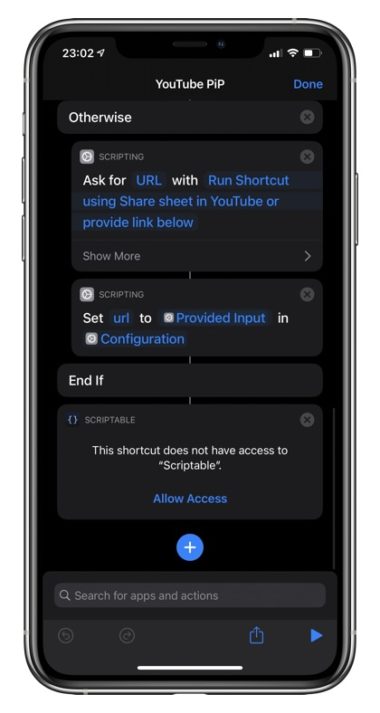The image showcases a smartphone with a sleek silver-gray frame. Along the left-hand side of the device, there are three visible buttons, while the right-hand side features a single button. The screen is predominantly dark with a black background. In the upper left-hand corner, the time is displayed in white as "23:02," alongside an arrow pointing diagonally to the right. The signal strength icon indicates good reception with three out of four bars filled in gray, and the Wi-Fi icon is fully illuminated in white, suggesting a strong internet connection. The battery icon, partially white, shows approximately 50% charge.

Below the status indicators, the screen displays a sequence of text and buttons. A line of white text reads "U2 PIP," with a blue "Done" button on the upper right-hand side. Beneath this, a dark black oval box contains the word "otherwise" in white text, followed by an "X" on the right side.

Continuing down, another box contains various script options. It reads "Script" in white, followed by "ask for" in white, then the blue text "URL." The script continues with the instructions in white, "run shortcut using share sheet in U2 but provide link below," ending with "show more" in white.

Further down, there is an additional script box that says "Script" in white, followed by "URL" in blue, then "to" in white, "provide input" in blue, "end" in white, and "configuration with an X" in blue.

Finally, the screen displays a line stating "end if" in white, followed by another message in white: "Scriptable, which is shortcut, does not have access to Scriptable," with a blue "Allow Access" option beneath it.